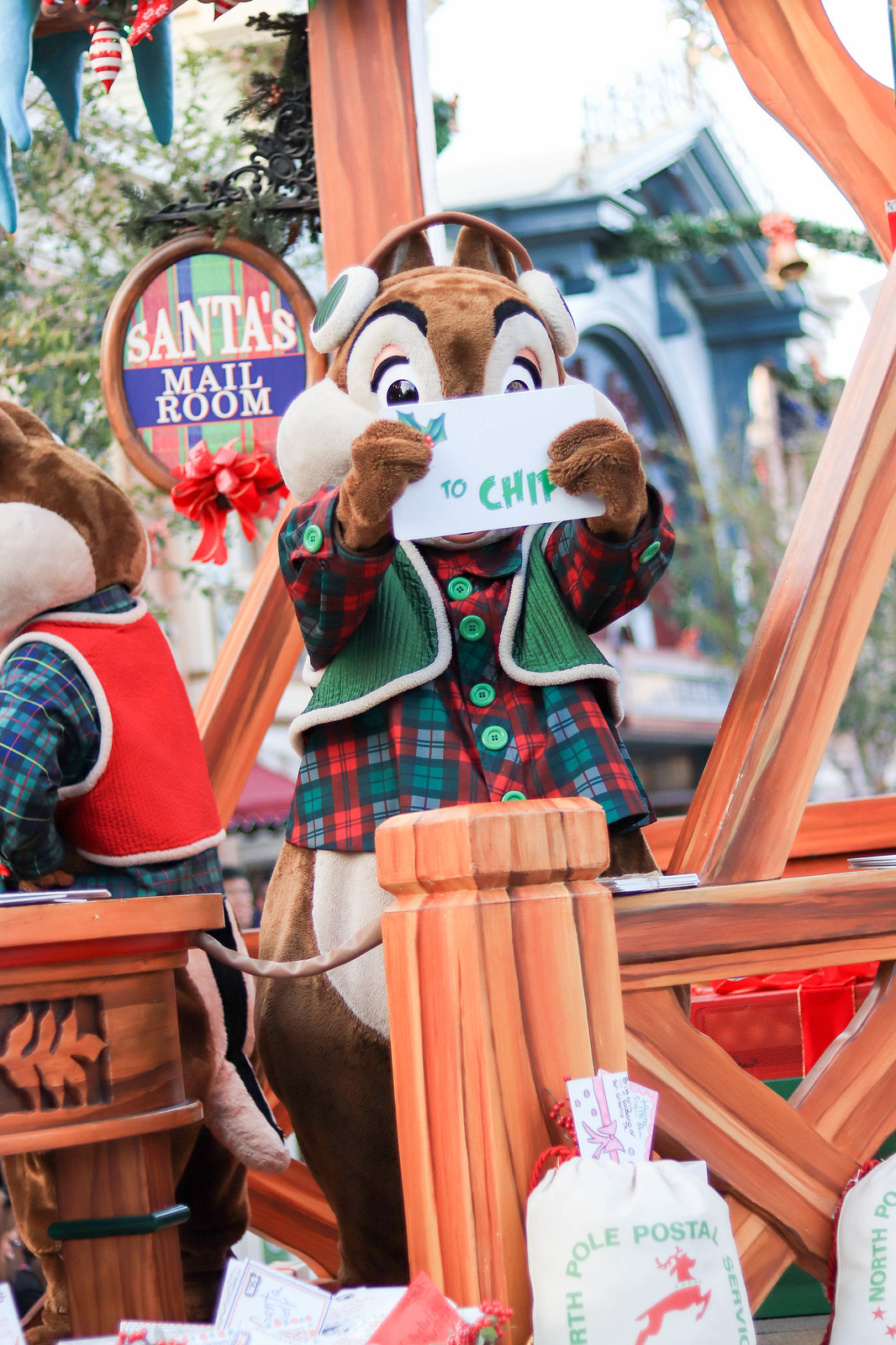The image depicts a festive Disney Christmas parade float themed as Santa's mailroom. Central to the scene is a costumed character, resembling either Chip or Dale of the Chip 'n' Dale duo, dressed in a Christmas-themed outfit that includes a padded green vest over a red, green, and blue checkered shirt adorned with large green buttons. The character is also wearing green earmuffs lined with white fur. The character holds a white envelope emblazoned with "To Chip" in green font, decorated with holly on one corner. Surrounding the character are various details contributing to the holiday atmosphere: mail bags labeled "North Pole Postal Service" with reindeer motifs strewn across the wooden floor, and another chipmunk mascot in a similar outfit positioned slightly behind and turned away from the camera. A prominent sign reading "Santa's Mail Room," embellished with a large red ribbon and holly, hangs from a wooden post, anchoring the scene’s festive decor. The background, though slightly blurred, reveals additional holiday decorations such as green wreaths and bells, with hints of buildings and trees completing the outdoor setting likely within a theme park like Disneyland or Disney World.